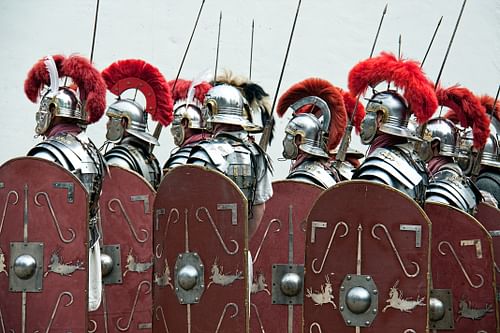This detailed photo captures a side view shot of a group of about eight or nine medieval soldiers, resembling gladiators or Trojan warriors, standing in formation. They are adorned in full silver armor, including helmets with distinctive red plumes that extend from the front to the back in a mohawk-like fashion. Each soldier holds a long pike pointed upward and carries a substantial reddish-brown shield, which features a prominent silver button or decorative circle in the center. Some shields also have additional silver studs around the edges, enhancing their ornate appearance. The soldiers are all facing left against a muted white or gray backdrop, presenting a striking and disciplined battle-ready scene.